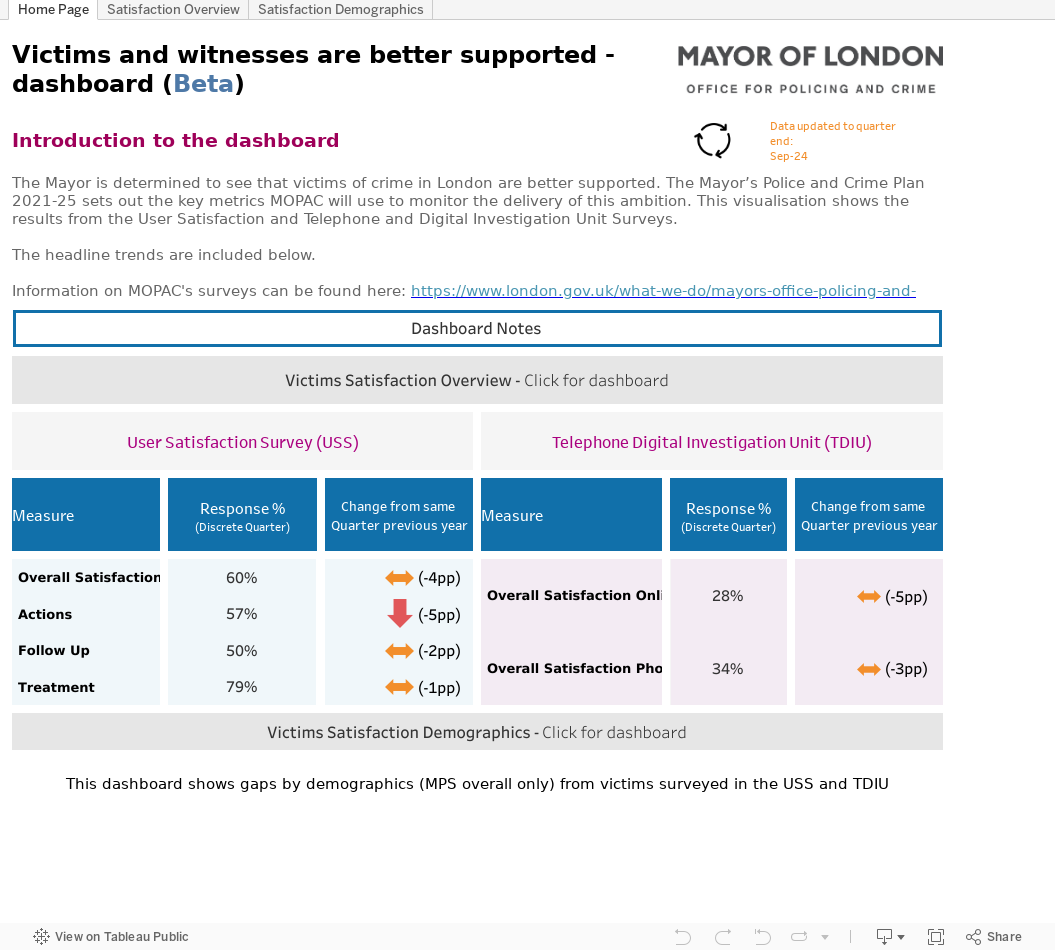In the image, we see a webpage designed for a computer display. At the top of the page, a header includes three tabs: "Home Page," "Satisfaction Overview," and "Satisfaction Demographics." Beneath this header, there is a prominent black-font title that reads "Victims and Witnesses are Better Supported Dashboard."

On the right side of this title, the text "Mayor of London, Office for Policing and Crime" is displayed. Just below, written in a purplish-pink font, there is an introductory paragraph about the dashboard. 

Scrolling down, towards the bottom of the page, we encounter a section titled "Victims Satisfaction Overview." This section features six columns, each with headlines highlighted in bright blue. The columns contain various statistics, including response times, measures, and changes from the same quarter of the previous year. Two of the columns are marked with yellow arrows, which likely indicate specific data points or trends.